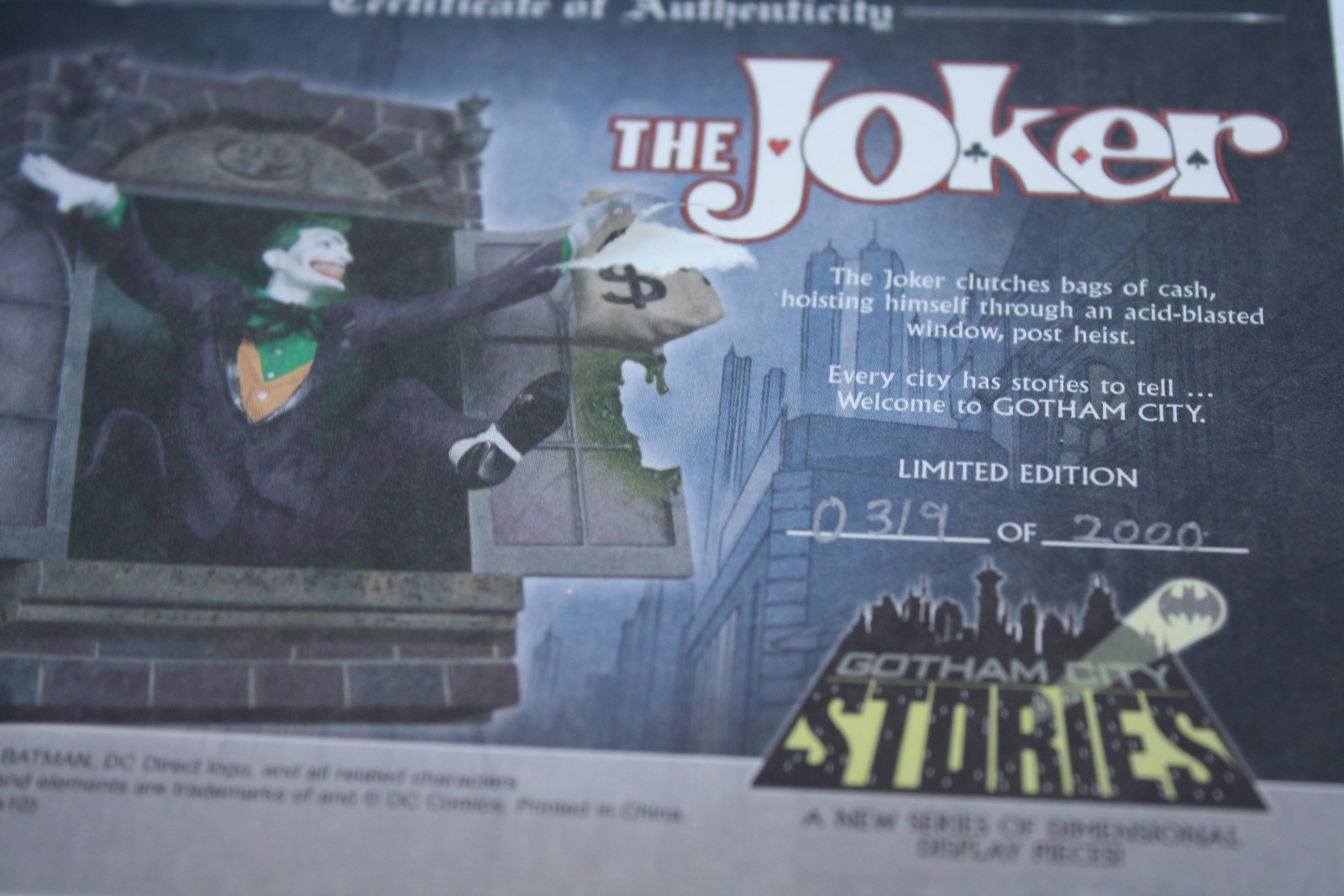This detailed image features a Certificate of Authenticity for The Joker, presented in a landscape-oriented, color photograph of a graphical illustration. Dominating the left side of the image is an intricately designed depiction of The Joker, emerging triumphantly from a shattered, acid-blasted window of a Gotham City building. Mid-heist, he clutches bags of cash and displays his signature sinister smile. Attired in his iconic purple suit with white gloves, black shoes, a gold waistcoat, a green shirt, and a large green bowtie, he exudes his well-known chaotic charm. His pale white skin, green hair, and vivid red lips are sharply detailed. The right side of the image is occupied by the textual elements, including the bold headline "Certificate of Authenticity" followed by "The Joker". Below this, an explanatory text reads, "The Joker clutches bags of cash hoisting himself through an acid-blasted window post heist. Every city has stories to tell. Welcome to Gotham City." It also notes that this is a Limited Edition item, numbered 0319 out of 2000. The background imagery features a dark, foreboding Gotham City skyline in blues and blacks. At the bottom right corner sits the "Gotham City Stories" logo, complete with the iconic Batman spotlight projected into the sky, encapsulating the gritty, narrative essence of the scene.